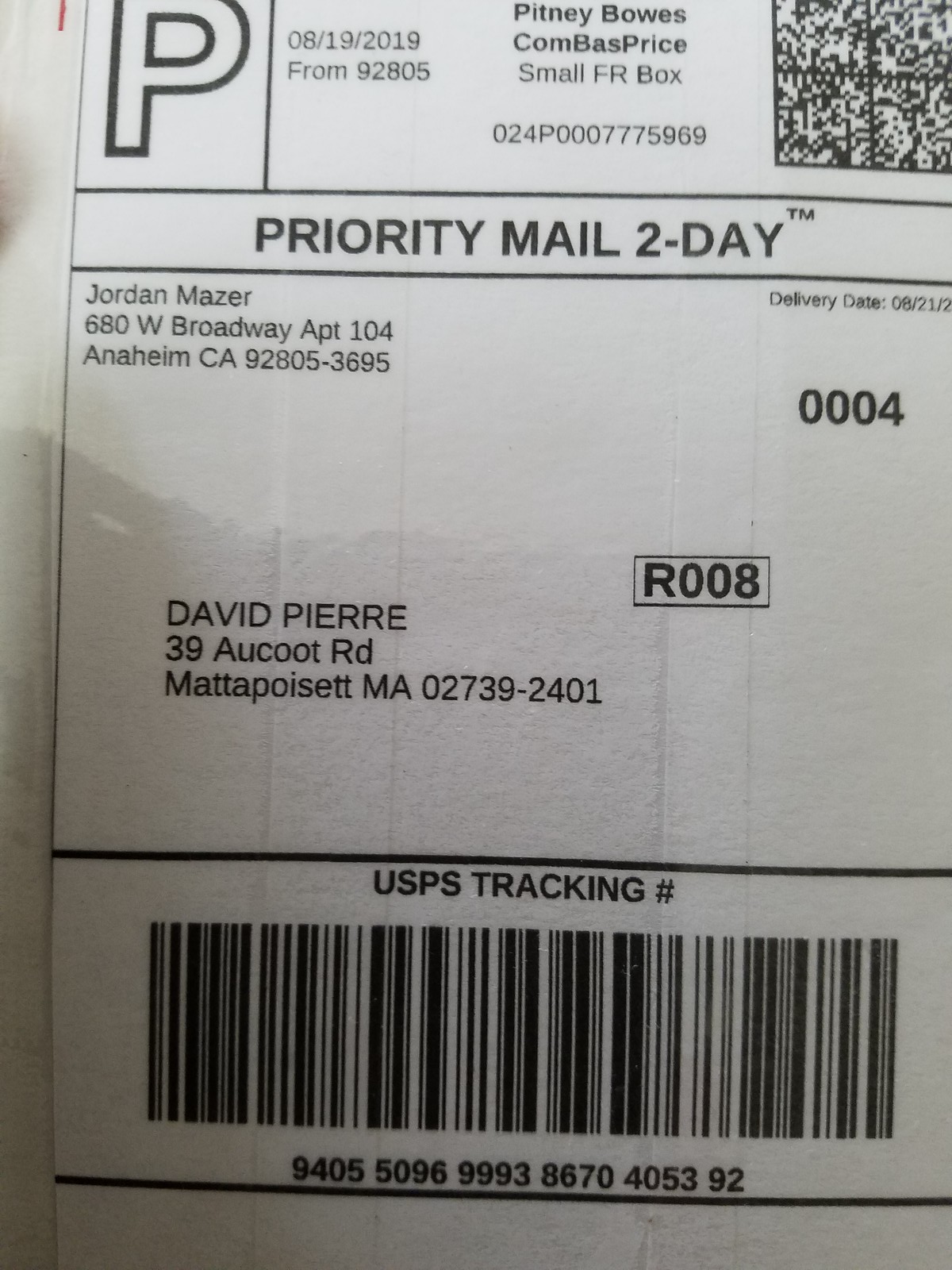The photograph is a colored image, despite its predominant black and white appearance, capturing a detailed USPS Priority Mail 2-Day shipping label. The label displays an issue date of August 19, 2019, and prominently features the sender and receiver information. The sender, Jordan Mazur, is located at 680 West Broadway, Apartment 109, in Anaheim, California. The package is addressed to David Pierre at 39 Aucout Road, Mattapoisette, Massachusetts, ZIP code 02739-2401. The label includes a black text on a white background, identifying Pitney Bowes as involved in the shipment. Below the recipient’s address, there is a barcode and a USPS tracking number: 9405-5096-9993-8670-405392.